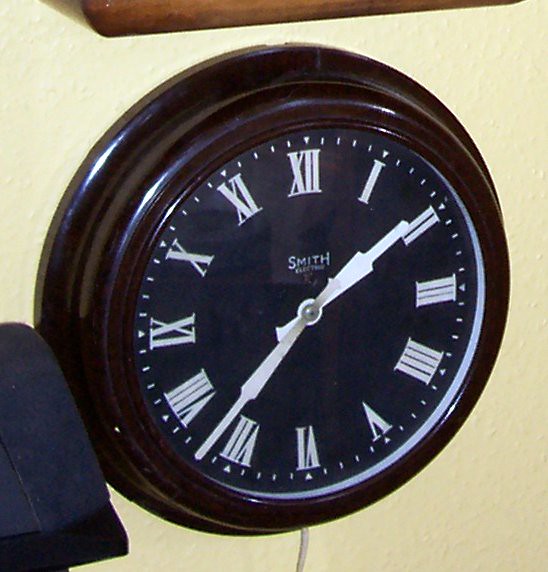The image features a close-up of a classic, wall-mounted, circular clock. The clock's frame is crafted from dark cherry-colored wood, possibly mahogany or dark walnut, lending it a rich, elegant appearance. The clock face itself is a deep, charcoal black and is adorned with off-white Roman numerals and minute markings around its circumference. The clock’s hands, including the second hand, are white to match the numerals and stand out distinctly against the dark background.

At the top center of the clock face, the brand name "Smith" is visible, although the second word is too small to be clearly read. The clock is powered by electricity, as evidenced by a white cord extending from the bottom, just below the 6 o'clock position.

The clock is mounted on a very pale yellow or cream-colored wall. Partially visible above the clock is the bottom edge of another wooden-framed item, possibly a picture frame or shelf, in a similarly dark wood. To the left of the clock, a piece of blue denim fabric is noticeable, adding a casual touch to the composition. The time displayed on the clock appears to be around 1:37.